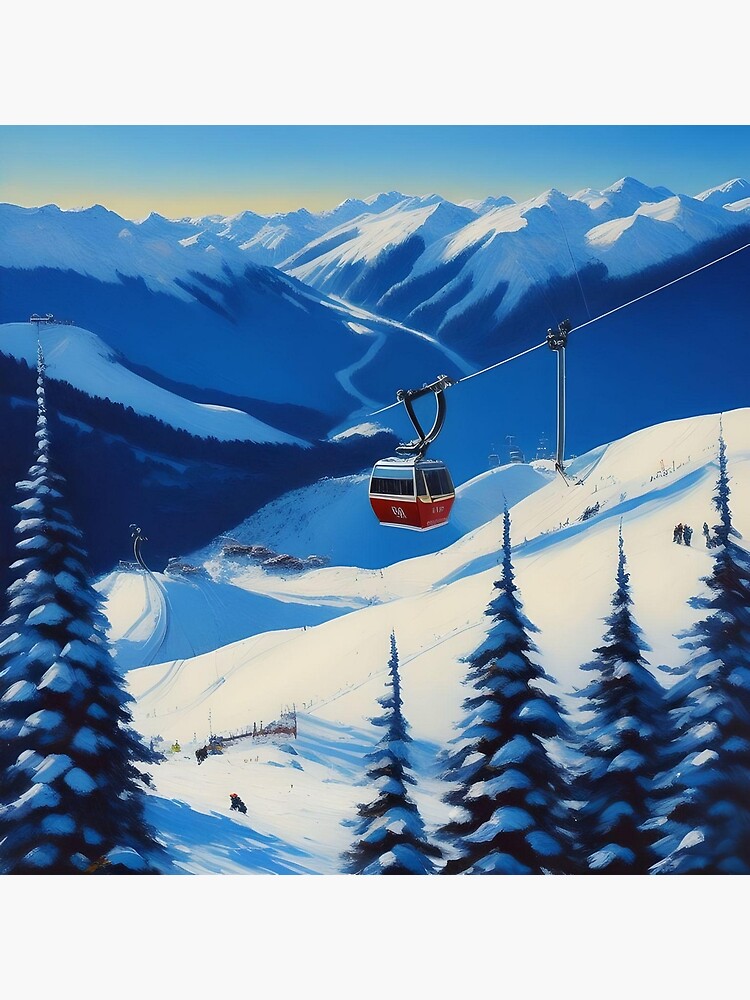The illustration is a square digital art print set against a white background, capturing a winter scene in vivid detail. Central to the image is a large, two-toned cable car, red at the bottom and black at the top, adorned with white markings and encased in windows. The car is part of a ski lift system, visibly linked to a metal pole and a zipline that extends diagonally upwards from the center out to the right.

Below the cable car, conifer trees blanketed in snow dominate the bottom of the image, with five tall trees prominently lining the foreground. The ground beneath them is a series of rolling, snowy hills that seamlessly blend into an expansive backdrop of snow-capped mountains. The peaks transition from a blue base to pristine white summits, creating a majestic mountainous landscape.

Scattered throughout the snowy terrain are small human figures, depicted in clusters or ascending the snowy slopes, adding a sense of scale and activity to the winter setting. The top of the image features a strip of blue sky, with a touch of yellow on the left, enhancing the picturesque, postcard-like quality of the scene.